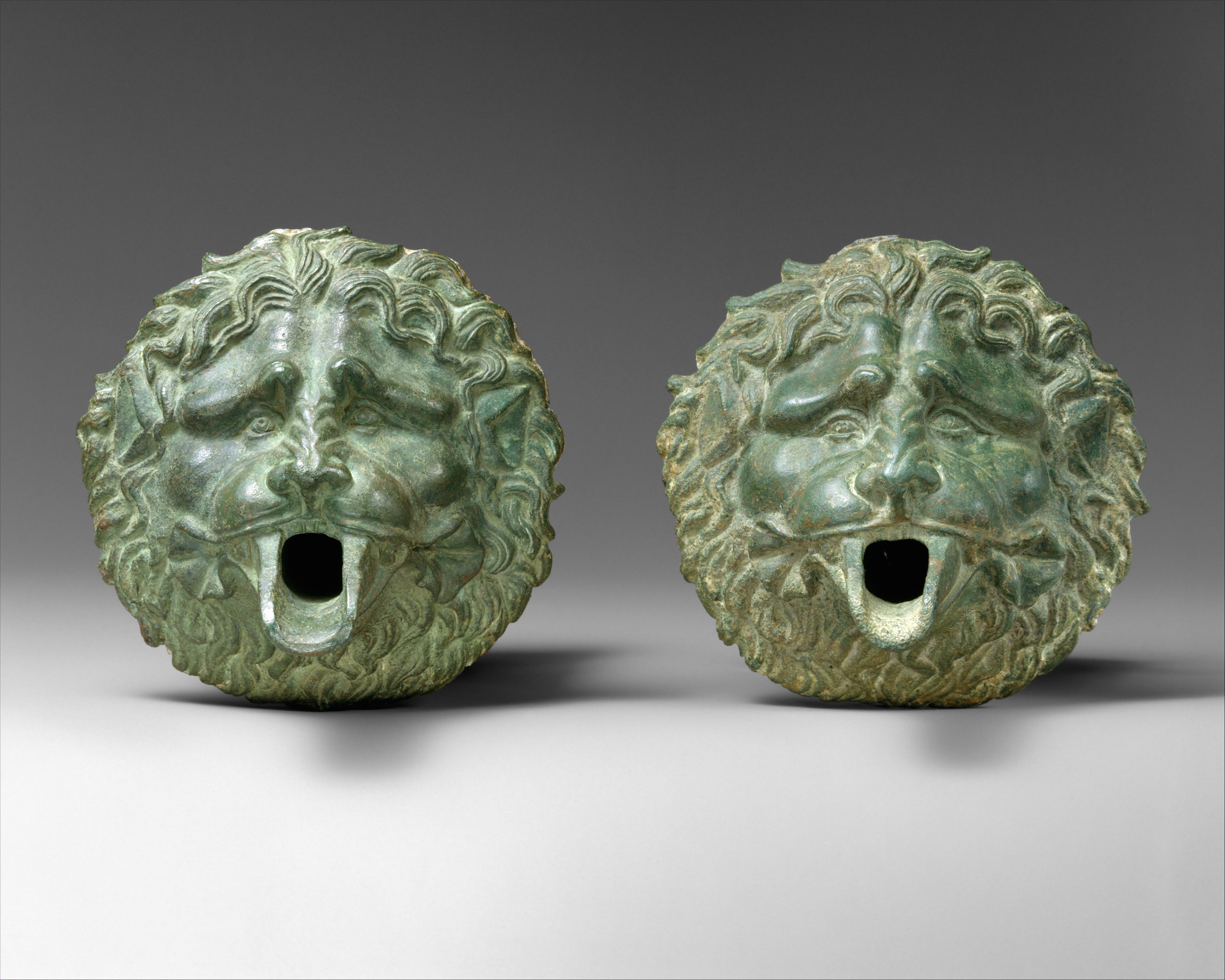This horizontal rectangular color photograph shows two nearly identical sculptures positioned on a plain gray platform, set against a medium gray background. The sculptures, which appear to be crafted from oxidized bronze, exhibit a greenish hue with hints of light brown or gold tint. Each sculpture features the face of a lion with distinct human-like attributes, including curly, almost circular hair resembling a lion's mane, expressive thick, curly beards, and prominent noses. The open mouths of the lions double as spouts, suggesting these could be intricate water fountain heads, similar to those found in Italy, designed to pour water straight down into a pool below. The precise context of their use is unclear, but the detailed craftsmanship and aged appearance suggest a historical or artistic significance, possibly photographed in a museum setting.